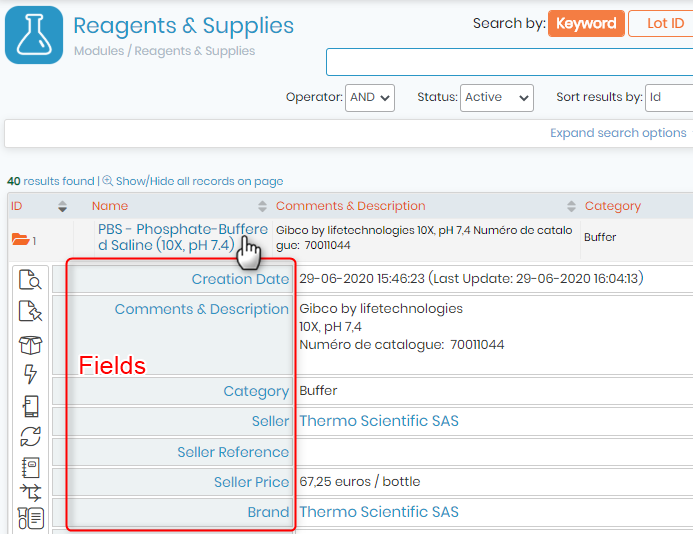The image depicts a detailed page from "Reagents and Supplies," showcasing a catalog or inventory system presumably used for scientific or medicinal purposes. The page prominently features a list with extensive information, highlighted by a red outline emphasizing key fields. These essential fields include Creation Date, Comments and Description, Category, Seller, Seller Reference, Seller Price, and Brand.

The first product listed bears the scientific name "PBS Phosphate Buffered Saline," indicative of its use in scientific applications. Further comments, written in technical language, accompany the product. 

At the top of the page, there are several functional tools for managing the inventory: a search bar allowing for queries by keyword or lot ID, selectable operators for refining searches, a status indicator (currently marked as active), and sorting options to organize results by ID. This comprehensive layout underscores the methodical organization and detailed nature of the inventory system, essential for scientific or medicinal supply management.